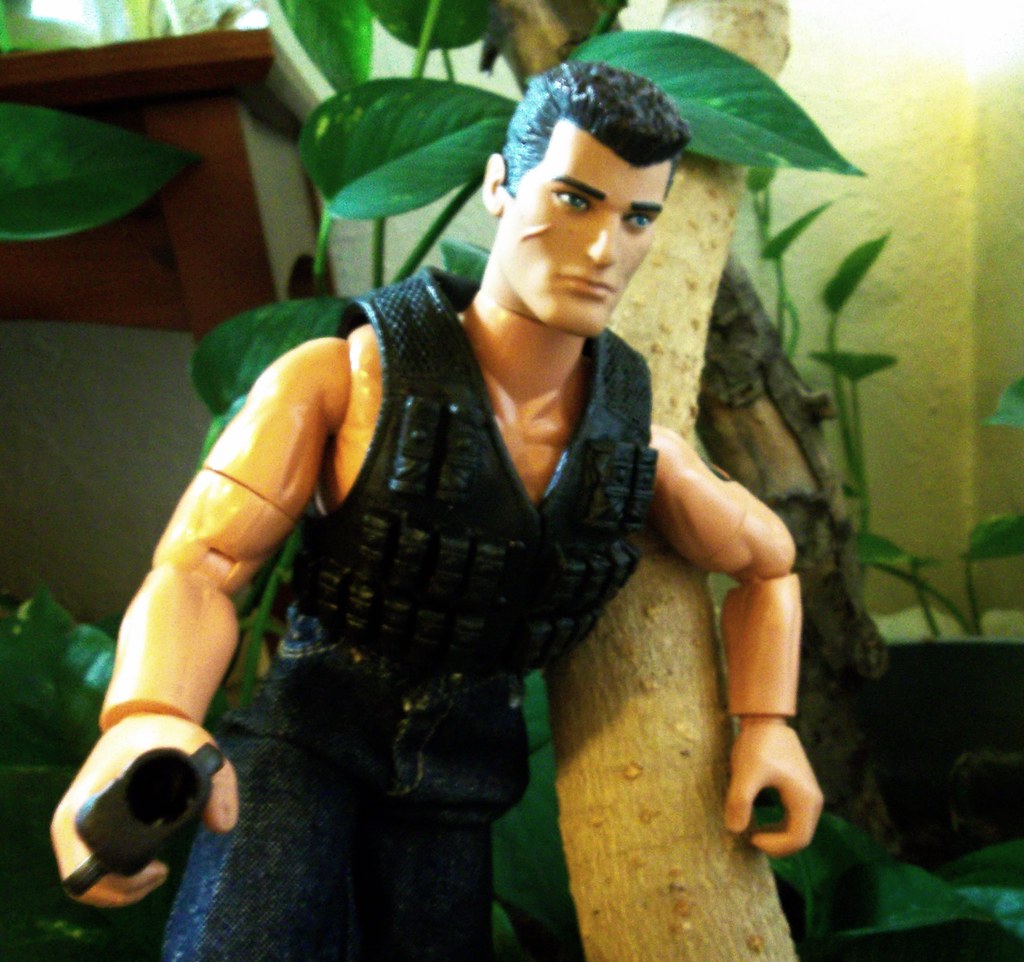A close-up photo captures a detailed action figure resembling a modified Ken or G.I. Joe doll posed in a miniature environment. The figure is outfitted as a tough military man, featuring a black sleeveless vest over his bare torso, blue jeans, and bendable arms that can detach at the biceps. His short brown hair is slicked back, and a prominent scar marks his right cheek. The doll's right hand clutches an object that appears to be a weapon. Positioned within what seems to be an aquarium or a potted plant setup, the backdrop includes branches, green leaves, and some wooden elements. The environment hints at a room corner, with light off-white stucco walls adding to the indoor setting. The lighting shines on the figure's right side, enhancing the detail of his rugged expression.